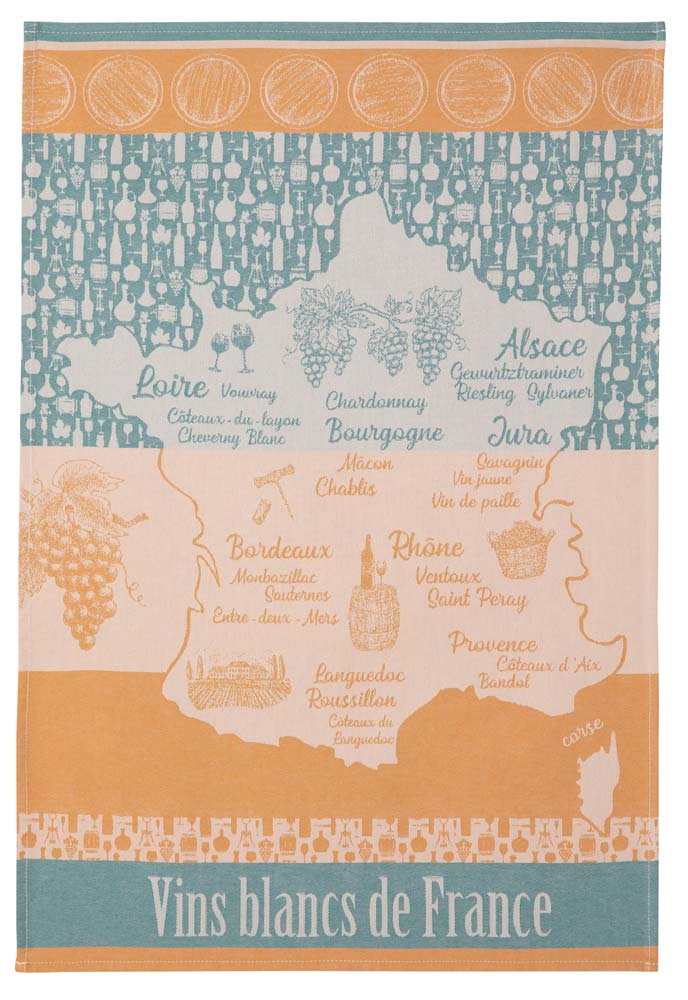This image is a detailed, colorful drawing of a map of France, showcasing its various wine regions and the specific white wines produced there. The map forms the central focus, with names of wines such as Loire, Vouvray, Chardonnay, Bourgogne, Alsace, Gervitz, Riesling, Sylvaner, Jura, Sauvignon, Ventoux, Saint-Péray, Provence, Coteaux d'Aix, Bordeaux, Languedoc-Roussillon, and Sauternes clearly labeled in their respective locations. The text is in French and serves to pinpoint the specific regions and wineries.

Surrounding the map are multiple colorful bands: a green band, an orange band with circles resembling the ends of barrels, another green and white band featuring wine bottle illustrations, a pink band adorned with grape graphics, an orange band with depictions of wine glasses and boxes, and finally a blue band with the text "Vingt Blanc de France." 

The overall color scheme incorporates robins-egg blue and creamy gold hues, creating a visually engaging contrast against a white background. Outside the map's outline, the top section displays images of various wine glasses and bottles in negative space, while the bottom is highlighted by a solid gold line. This artistic representation could be part of a magazine cover or even designed on fabric, offering a lively, informative guide to France's celebrated white wines.